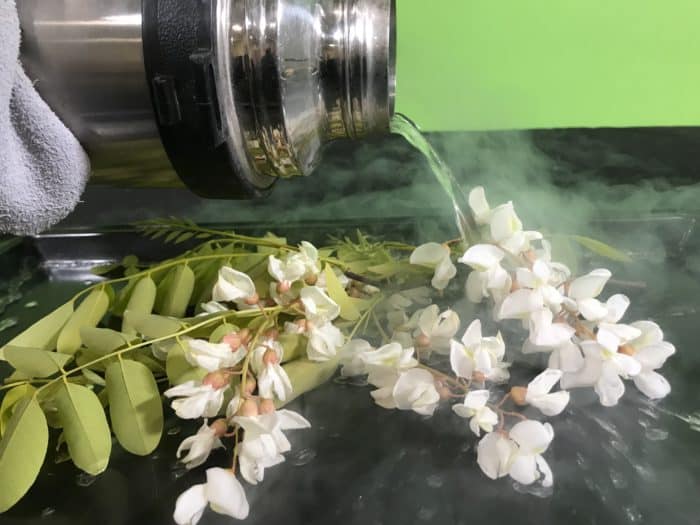In this photograph, white flowers with green stems sit on a dark, possibly black or metallic base, situated in the center of the image against a vivid green background. A person, partially visible, with a blue towel or grey glove around their hand, holds a shiny metal thermos or canister to the left of the frame and pours a clear, steamy liquid over the flowers. The liquid produces a significant amount of steam, suggesting it could be extremely hot or possibly a substance like liquid nitrogen. The scene is quite moody and reflective, with the precise nature of the liquid and the intent behind the action remaining ambiguous.